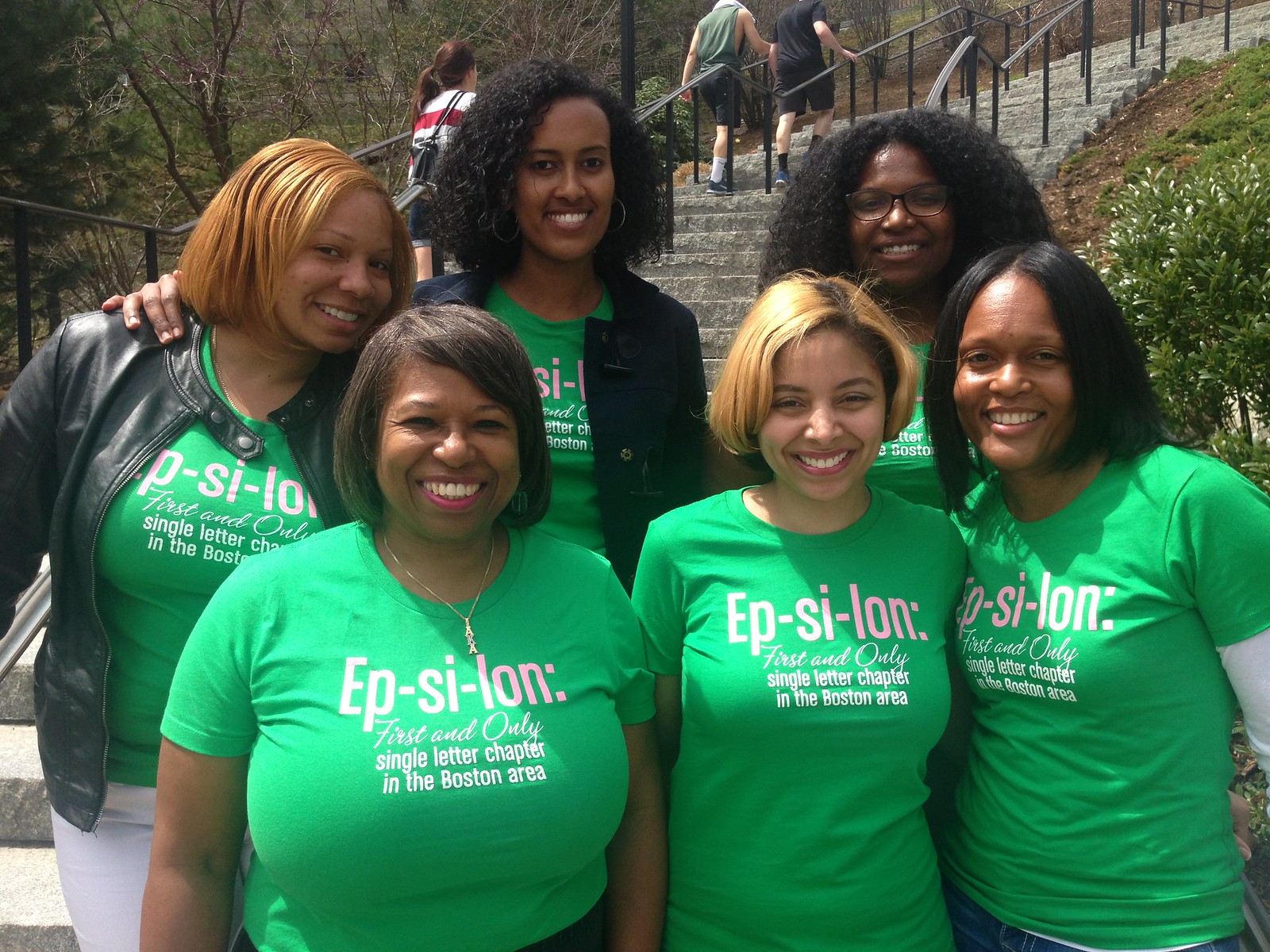The image features a group of six African-American women, all proudly wearing short-sleeved, bright green shirts emblazoned with "EPSILON" in dashed white letters, followed by the phrase "first and only single letter chapter in the Boston area" in smaller text. They are gathered outdoors in front of a set of stone stairs with black handrails, which ascend a steep hill. This could suggest a college campus setting. The background includes trees and greenery, with a green bush visible to the right of the group. A couple of other individuals are seen walking up the stairs in the background. The group consists of three women in the back row and three in the front row. The women in the back left are wearing black jackets over their green shirts. The back row includes a woman with dark blonde hair, a woman with black curly hair, and a woman with glasses and black curly hair. The front row includes a woman with short dark hair, a woman with a pixie cut and dark blonde hair, and a woman with shoulder-length black hair. All of the women are smiling warmly at the camera.